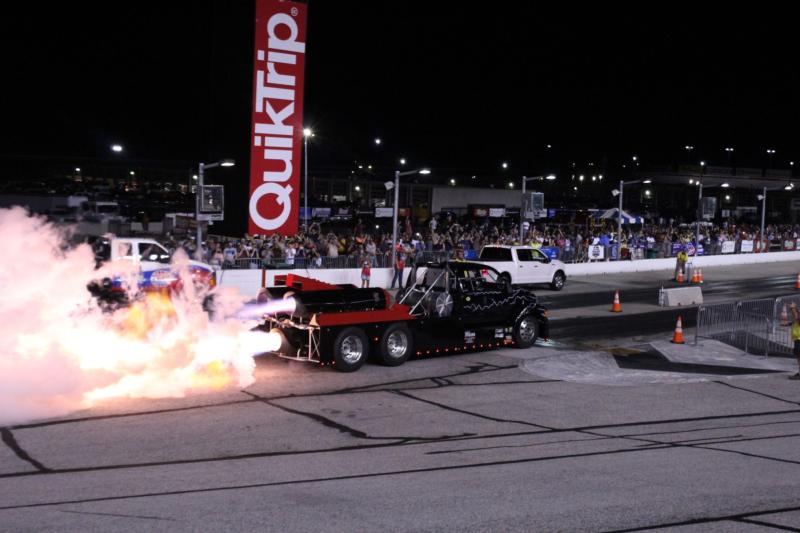In this image, a dramatic nighttime scene unfolds at a drag racing track, where a powerful flatbed truck equipped with three rocket engines is poised to take off, flames and thick smoke billowing from its rear. The black-and-red truck, sponsored by Quick Trip, is centered on the image, with a large red QT sign prominently displayed above. A brave individual stands at the starting line, ready to signal the start amid roaring engines, with minimal protection if something goes awry. In the background, packed stands are filled with eager spectators behind concrete and metal barriers, all under the dusky sky dotted with light posts. Two safety trucks, a pacing vehicle, and a rescue truck are visible, positioned for quick response. The track itself shows signs of wear, with tar-filled cracks and a light gray roadway visible at the bottom, flanked by traffic cones. The atmosphere is intense and electrifying, promising a loud, high-speed showdown.